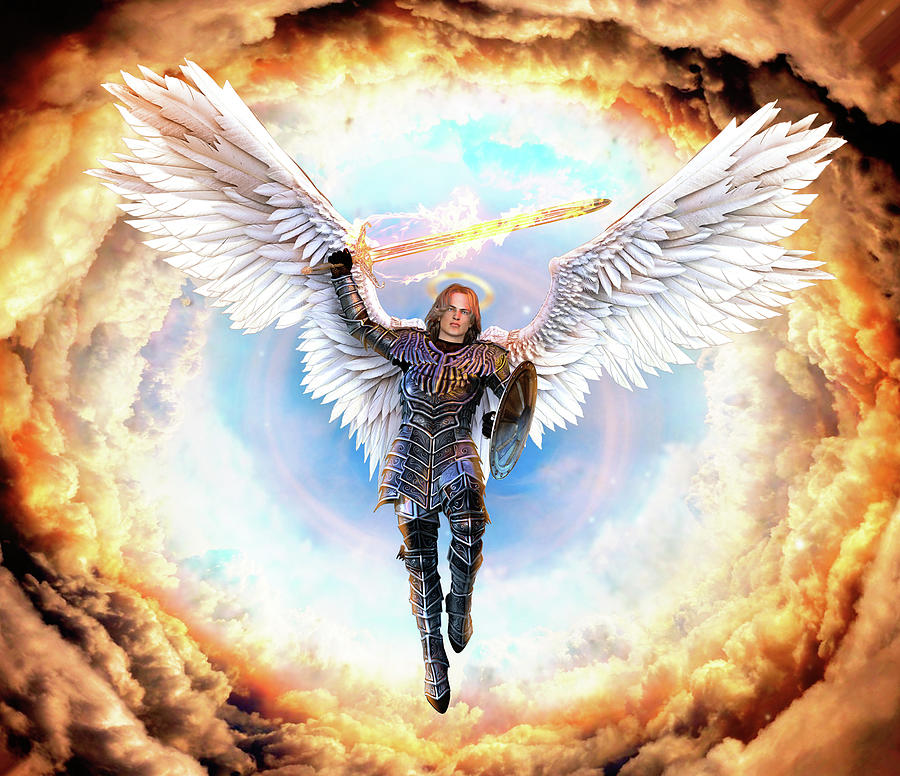This digital illustration depicts an angelic figure with long blonde hair cascading to their shoulders, clad in a full suit of metal armor including matching boots. The figure holds a round metal shield in their left hand and raises their right arm, gripping a glowing, fiery sword. Large, pristine white, feathery wings extend majestically from their back. A radiant golden halo hovers above their head. Surrounding the central figure is a dramatic backdrop of swirling orange and brown smoke clouds, forming a circular tunnel that frames the angel. Beyond these clouds, the sky glows a soft blue, highlighting the ethereal and otherworldly nature of the scene. The figure's gender is ambiguous, with some elements suggesting a possible homage to Joan of Arc.